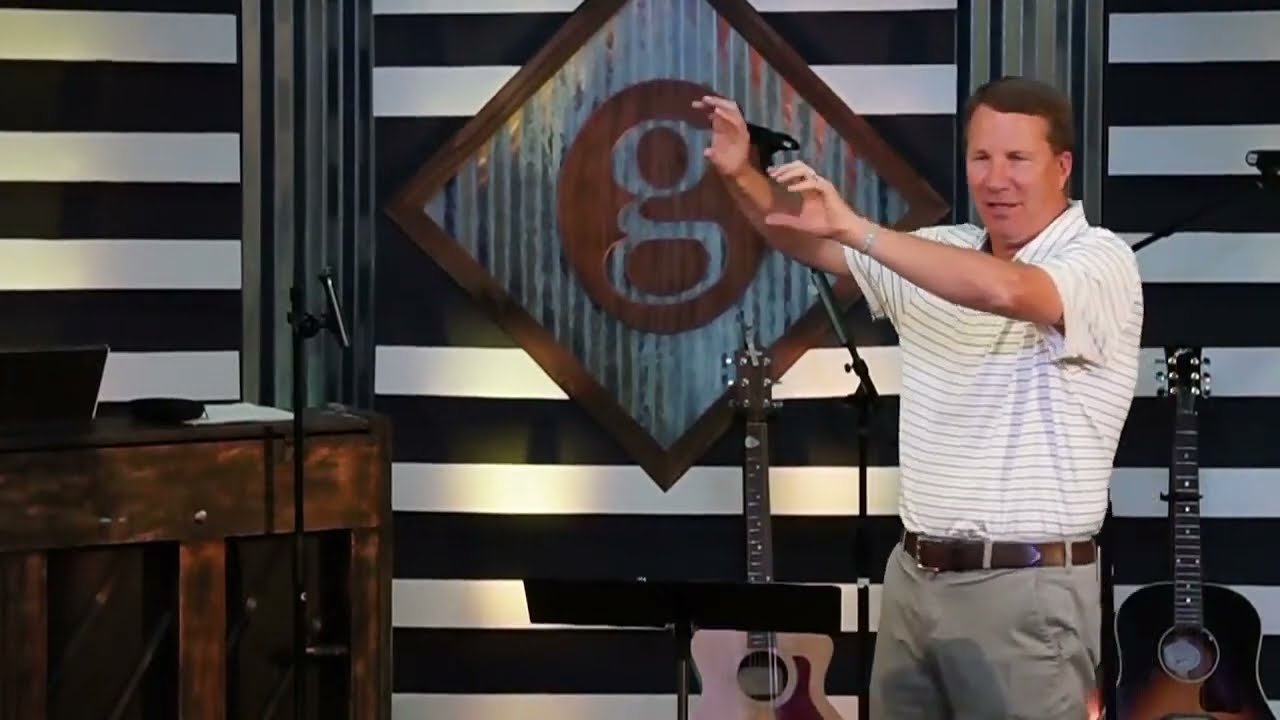In the screenshot, we see an older Caucasian male, likely an American in his 40s or older, positioned on the right-hand side of the image. He has short brown hair and is dressed in a short-sleeved white shirt with black stripes, tucked into grayish chino pants secured with a brown leather belt. He is wearing a silver bracelet watch on his left hand, and you can see the outline of a cell phone in his left pocket. His hands are raised near his face as if he is gesturing or explaining something.

The background features a modern black and white striped design with a diamond-shaped symbol containing a lowercase 'g'. Behind him stand three microphones and two acoustic guitars in their stands. On the left side of the image, there is a podium with a microphone, and in the background, a piano with a microphone on it can be observed. The scene appears to be set in a space possibly related to music or a concert, with elements hinting at it potentially being a venue for performances or even a sermon.